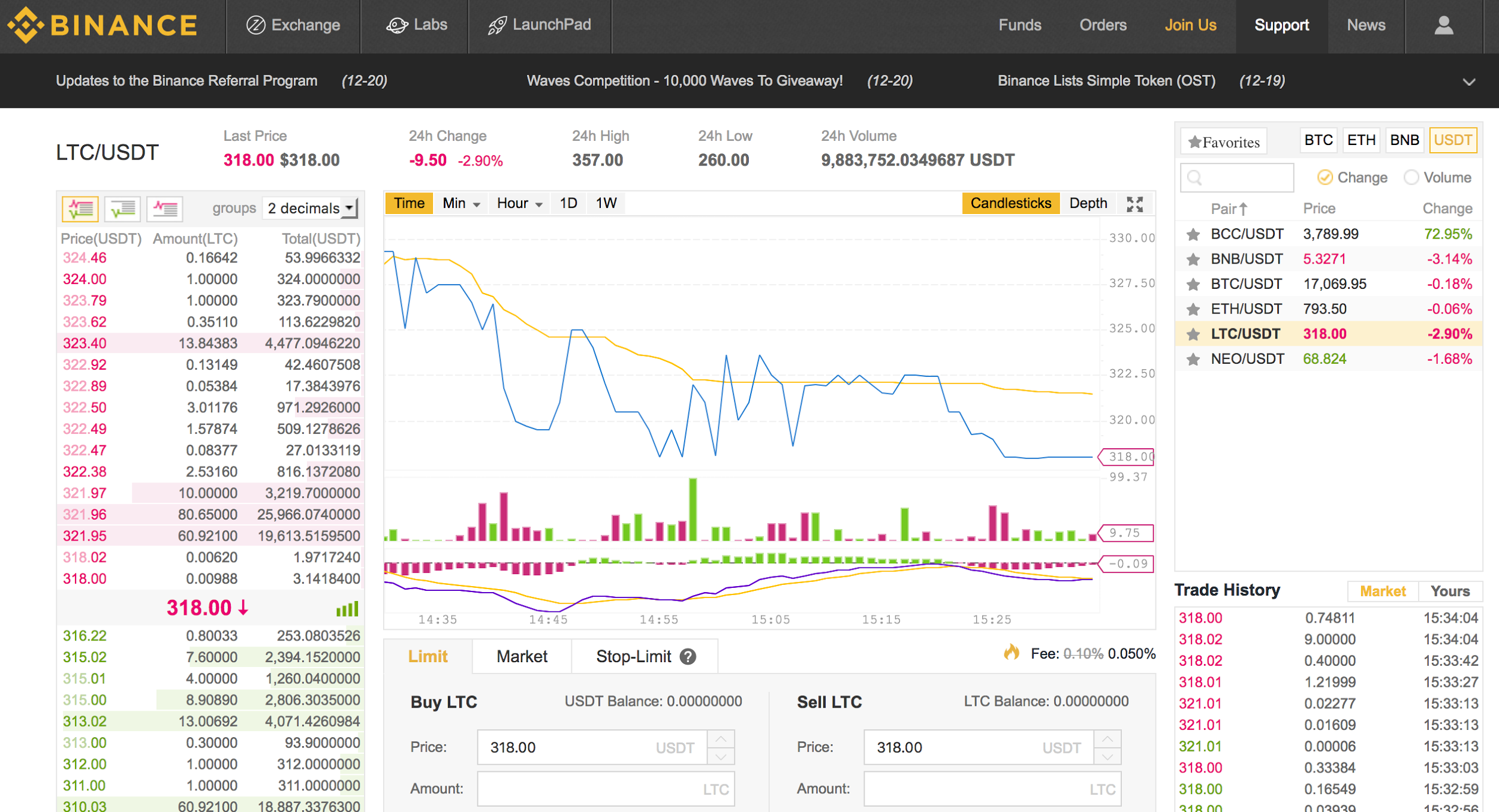The image captures a detailed interface of a cryptocurrency exchange platform, resembling a stock market dashboard. The left side of the graphic is populated with a plethora of numerical data associated with price, amount, and total, creating a comprehensive ticker-like display. At the very top, there's a main navigation bar that includes options such as "Exchange," "Labs," and "Launchpad," accompanied by additional tabs for "Funds," "Orders," "Join Us," "Support," "News," and an "Account" icon for user login.

Prominently, the header announces updates to the "Be Nice" referral program dated 12-20, and a "Wave Competition" with a giveaway of 10,000 waves also marked for 12-20. Mention is made of something titled "Lot Simple Token" dated 12-19, though this part is somewhat unclear.

Below the headings, there is a detailed price conversion section featuring LTC (Litecoin) and USDT (Tether), highlighting key indicators like the 24-hour range, 24-hour high, 24-hour low, and 24-hour volume. The right side of the interface showcases a customizable list of favorite trading pairs, facilitating quicker access. Users can filter this list based on changes and have options to include BTC (Bitcoin), ETH (Ethereum), BNB (Binance Coin), and USDT trades.

The bottom of the screen features trading options including "Limit," "Market," and "Stop Limit," along with buttons for buying and selling LTC. It specifies the fee percentage for trades and includes a trade history section on the bottom right corner, allowing users to keep track of their market activity. The left side displays a list of various cryptocurrencies, each annotated with their current status, such as one marked as down by 318 points, helping users quickly assess market conditions.